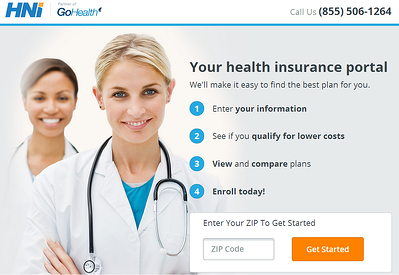The webpage features a streamlined design focused on health insurance services. At the top, there's a clean banner with "HNI Go Health" prominently displayed in blue lettering against a white background. To the left side of the banner, in black letters, it reads "Call Us" followed by the contact number of the health insurance provider.

In the main section of the page, two women dressed in hospital scrubs are prominently featured, symbolizing healthcare and support. To the right of this image, a bold heading reads, "Your Health Insurance Portal," accompanied by a subheading that encourages users with the phrase, "Make it easy to find the best plan for you." 

Below these headings, the page provides step-by-step instructions for visitors, beginning with a prompt to "enter your zip to get started." Directly beneath this text, there's a box for users to input their zip code, accompanied by a prominent "Get Started" button to the right, designed to guide users through the initial steps of finding their ideal health insurance plan.